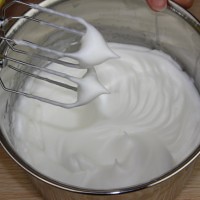This detailed square image captures a close-up view from a slightly elevated angle of a deep, silver metal mixing bowl—possibly aluminum or stainless steel—partially filled with beautifully whipped egg whites, forming soft peaks and smooth, fluffy layers reminiscent of meringue. Though the rest of the kitchen mixer isn't visible, two silver beaters with four prongs each are suspended above the bowl, still carrying some of the egg whites on their edges, hinting at the recent whipping activity. A thumb is subtly visible at the top of the frame, suggesting someone is holding the bowl steady. The setting features a brown background that appears to be a wooden counter.